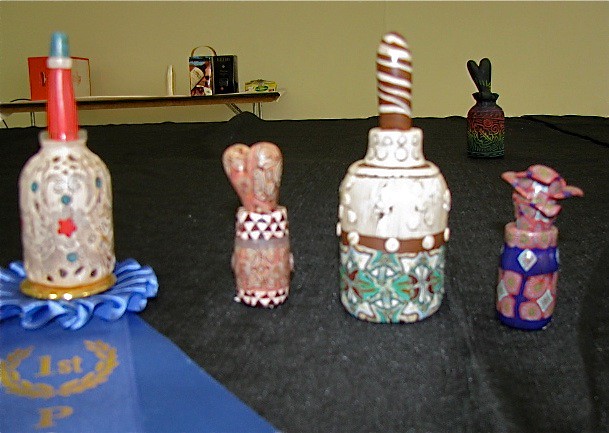This photograph captures a collection of intricately crafted glass and ceramic items, set upon a table draped in black fabric. In the leftmost corner, a blue section featuring a golden "First" and a Roman crown emblem stands out, attached to a blue ribbon signifying a prize winner. Directly beneath this ribbon is a white structure with a distinct red, bell-shaped handle, topped with a small blue tip.

To the right of this piece are several more unique items. The first is a brown jar with a prominent red neck, followed by a larger brown ceramic piece topped with a heart-shaped lid. Next, there is a white object adorned with circular protrusions, and a brown-and-yellow piece featuring an intricate handle design. On the far right, a small item showcases blue and pink colors with alternating white and black triangular patterns.

In the background, a second table holds an assortment of three boxes, and a colorful black figurine adds further interest to the scene. The wall behind these tables is painted beige, providing a neutral backdrop that emphasizes the vibrant and varied colors of the items on display.